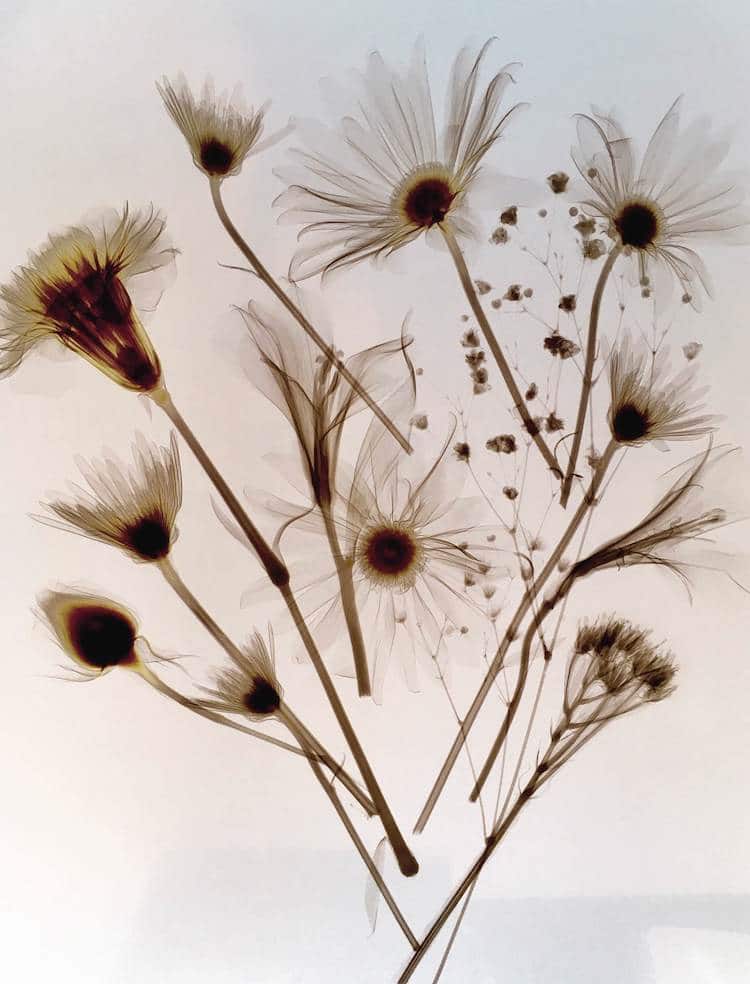This photograph presents a close-up of a bouquet-like arrangement of roughly ten white flowers, resembling daisies. The flowers, which appear either suspended or laid on a white surface, possibly dried and pressed like those you would find in a book, are captured in a light sepia or black-and-white, x-ray-like style that inverts their natural colors. Each flower displays numerous, semi-transparent petals with centers that transition from white to yellow to a burnt brown. The stems, a blend of brown and green, remain visible with their ends cut off. Among the flowers, some are fully opened, while others remain in various states of bloom, with some buds still closed. A few petals are broken and scattered around, and in the bottom right, a flower that never bloomed appears to have withered. The overall composition allows for an individual view of each flower, making the intricate details of their structure and the nuanced play of light and shadow strikingly apparent.